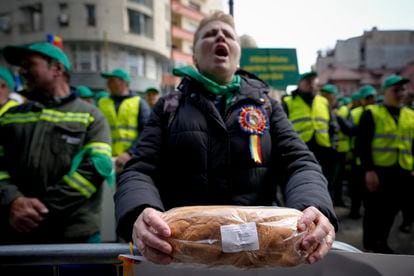In the lively scene, several men and women stand on the street in front of various buildings, all donning bright neon green safety belts and deep green hats. Their high-visibility vests reflect a sense of unity, possibly suggesting a collective action. Prominently positioned in the center is a person with short blonde hair, clad in a deep blue bubble winter jacket with a blue, yellow, and red ribbon pinned to it. This person, possibly yelling, clutches a large loaf of bread wrapped in plastic, symbolizing the economic struggles they are protesting against.

This evocative protest scene is reminiscent of the recent yellow vest demonstrations in France, where workers raised their voices against pension reforms and economic inequality. The green sign with yellow lettering in the background adds to the atmosphere of organized civil resistance. The group's stern faces and determined posture convey a powerful message of defiance and solidarity on the bustling city street.